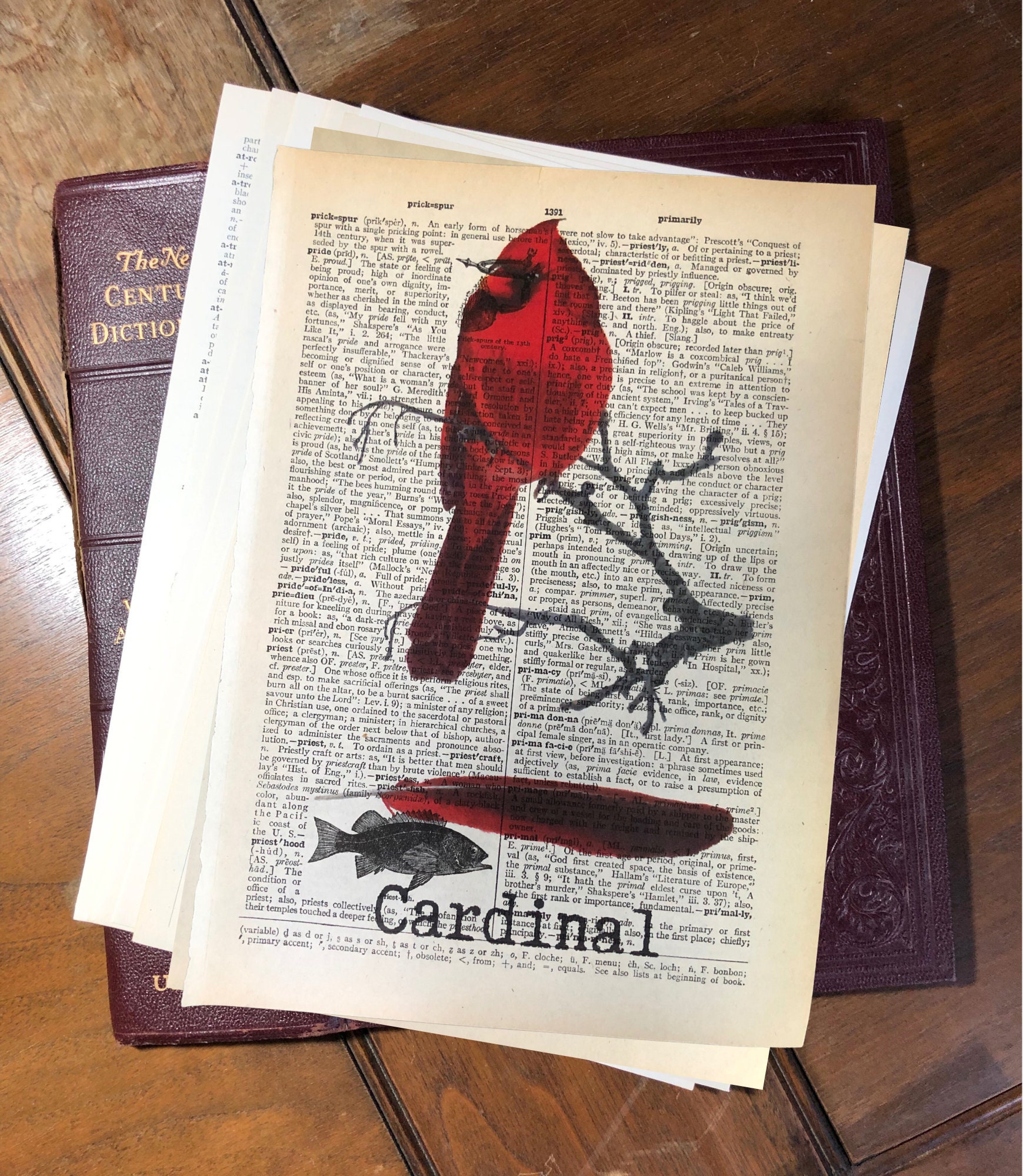The image showcases a detailed illustration of a bright red cardinal perched on a dark gray branch, overlaying a page from a dictionary. The dictionary page, along with a few other similar pages, is stacked atop a burgundy leather-bound dictionary, identified as "The New Century Dictionary." The pages are laid out on a wooden surface, which appears to be a table or floor. Below the cardinal illustration, there is a horizontally positioned red feather and the word "cardinal" prominently written in black text. Surrounding the illustrations are two columns of word definitions in black text, indicating the page's original function as a dictionary entry. The wood surface beneath the dictionary and pages features some engravings, adding texture to the scene. The small print on the dictionary pages likely provides details about the cardinal, its habitat, diet, and other pertinent information, although it’s too small to read clearly.